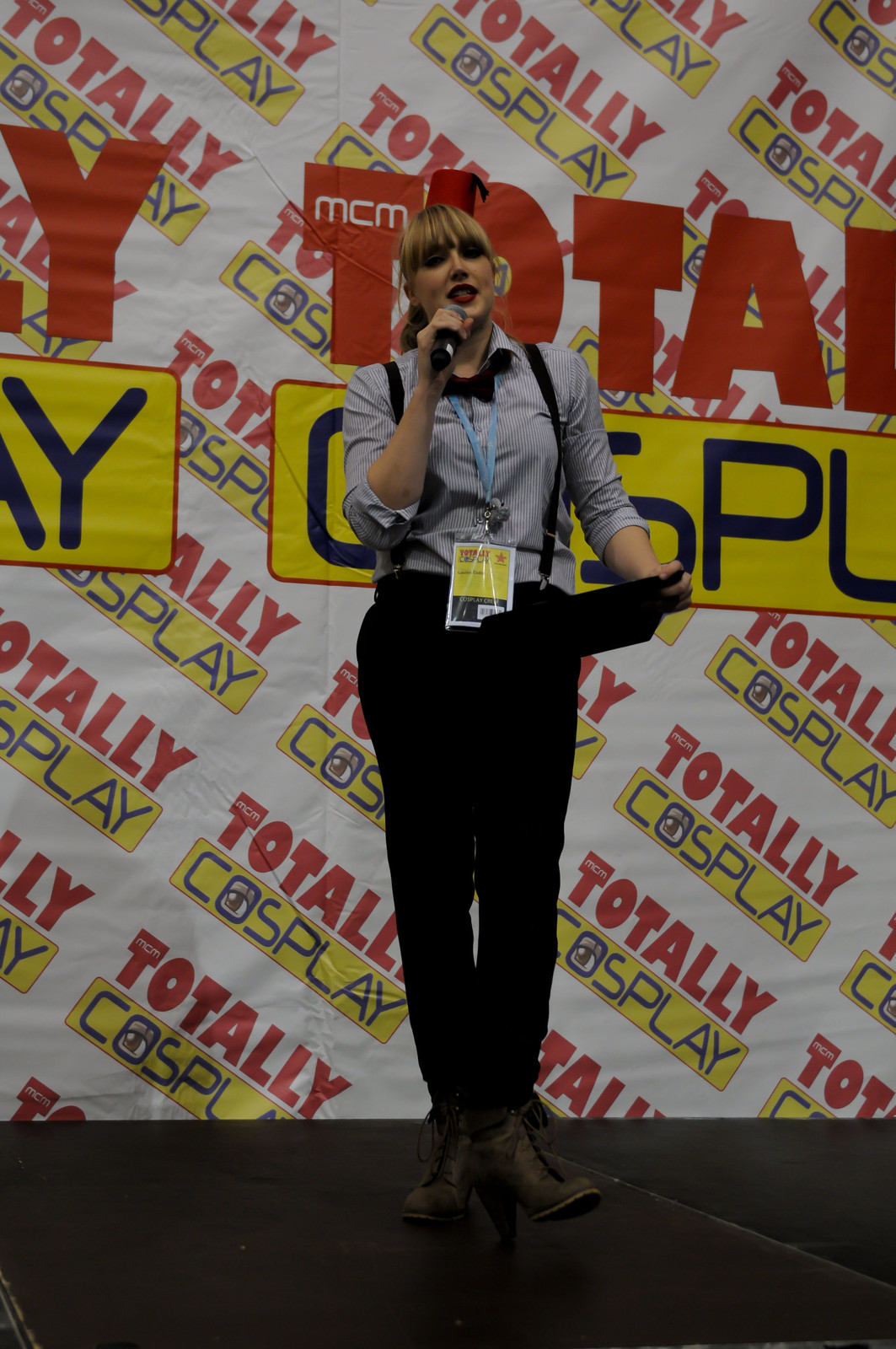The photograph features a young blonde woman standing on a stage, holding a microphone in one hand and what appears to be an iPad or a clipboard in the other. She stands before a backdrop adorned with large "Totally Cosplay" logos written horizontally across the center, and a pattern of smaller logos diagonally covering the entirety of the white background sheet. Dressed in black pants and high-heeled brown boots, she also sports a gray pinstripe button-down shirt with the sleeves rolled up to her elbows, complete with suspenders. Around her neck hangs a name tag on a lanyard, indicating her official role at the event. She appears to be either running the show or introducing acts, possibly serving as the master of ceremonies for the event.